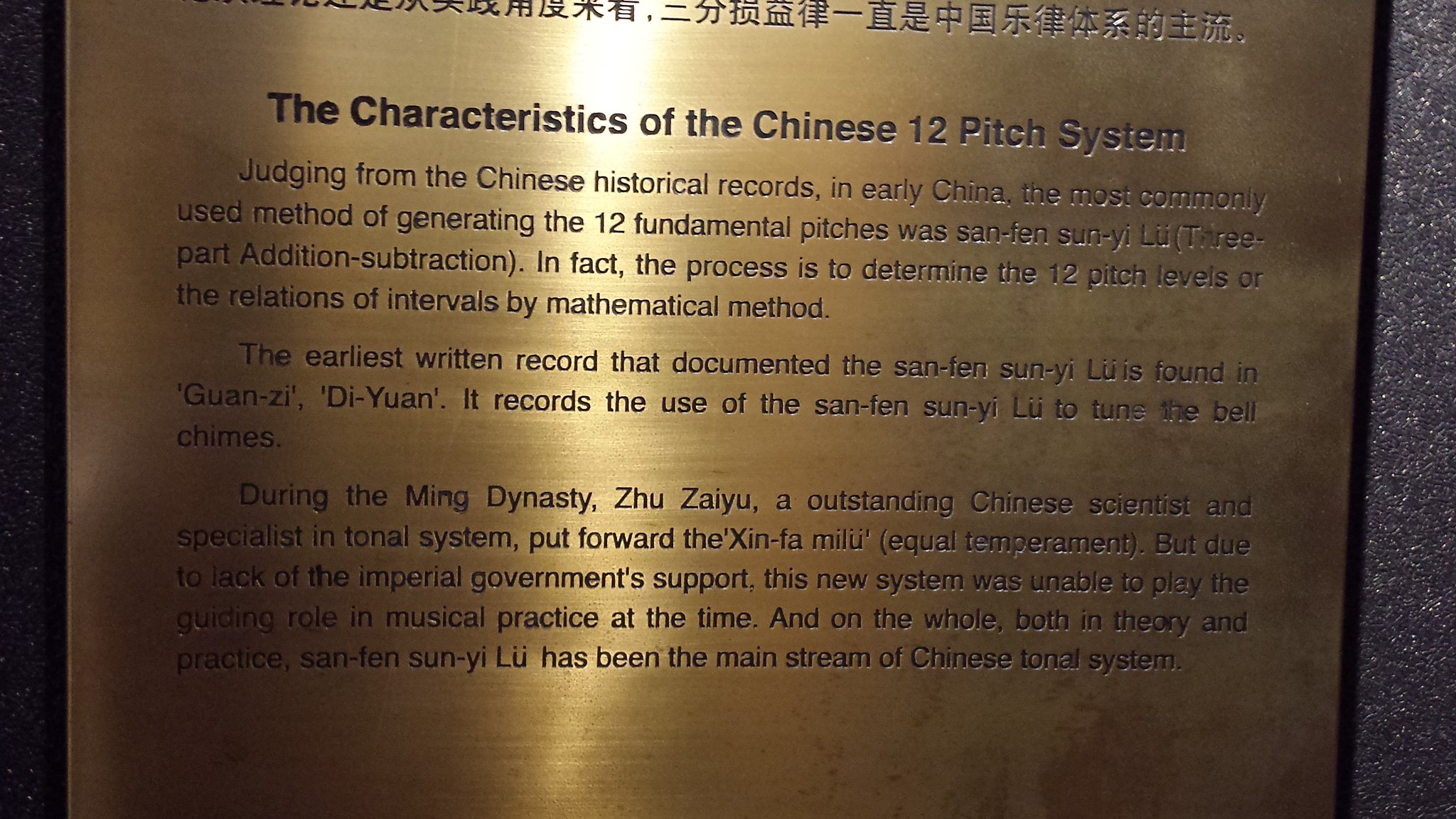The image is a color photograph in landscape orientation, featuring a bronze or gold-colored commemorative plaque that is partially cut off at the top and bottom. The plaque, set against a dark speckled granite background visible on the right side, includes black script and a heading that reads, "The Characteristics of the Chinese 12-Pitch System." Below the heading, there are three paragraphs of text detailing the historical method known as San Fen Sun Yi Lu (three-part addition subtraction) used in early China to generate the 12 fundamental pitches through mathematical methods. The earliest written record of San Fen Sun Yi Lu is found in the Guanzi Diyun, which mentions its use in tuning bell chimes. During the Ming dynasty, Zhu Zanyu, a prominent Chinese scientist and tonal system specialist, introduced the Zhen Fa Mi Lu (equal temperament). However, due to a lack of imperial support, this new system did not influence musical practice at the time. Overall, both in theory and practice, San Fen Sun Yi Lu has remained the mainstream of the Chinese tonal system.